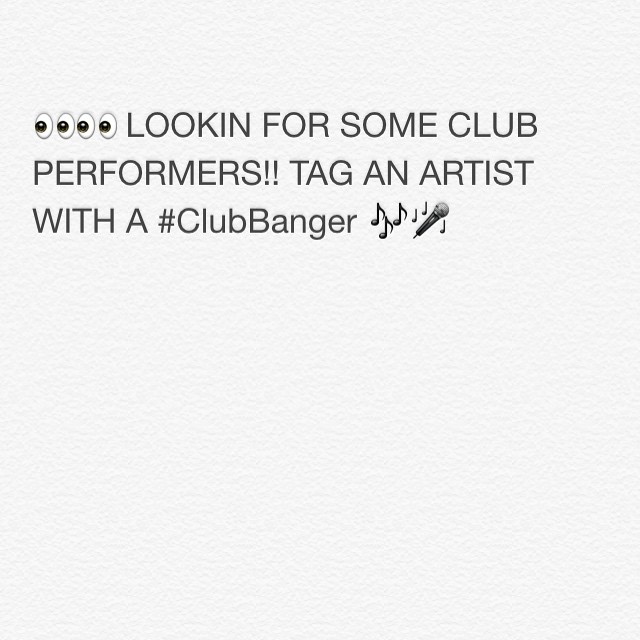The image is a simple, square advertisement with a textured, off-white background reminiscent of eggshell or pearl white. Positioned towards the top of the image is a block of plain black text in a casual, all-caps font. The text begins with four eye emojis that appear to be looking to the left. Following these symbols, the text reads "LOOKING FOR SOME CLUB PERFORMERS!!" The word "LOOKING" omits the "G" to enhance the informal tone. Below this, it says, "TAG AN ARTIST," accompanied by the hashtag "CLUB BANGER," which is not in all caps. This hashtag is flanked by several musical note emojis and a drawing of a microphone alongside another single musical note. The entire layout is clean, with no additional elements beyond the described text and emojis, suggesting it might be a screenshot from Instagram.